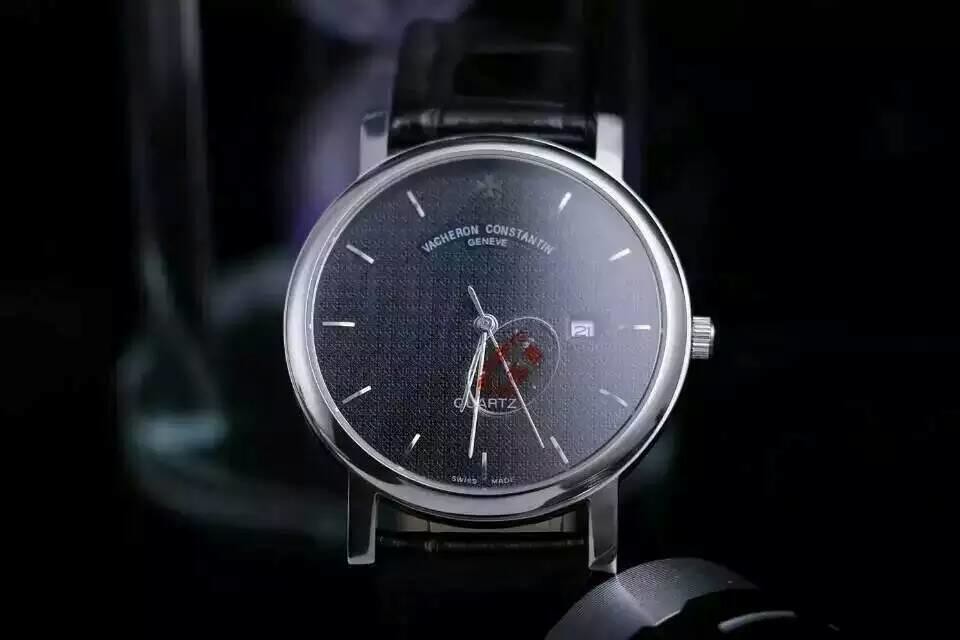This photo captures an elegant silver-framed quartz watch standing upright, with no wrist in sight. The watch features a black leather strap extending upwards and a round black face adorned with minimalistic white slashes instead of traditional numbers. Notably, the 12 o'clock position is marked with the head of a lion. The brand name "Vacheron Constantin, Geneve" is prominently displayed on the upper part of the dial, while "quartz" is inscribed below the watch hands. There's also a small window indicating the date as the 21st. The current time shown is just after 6:30, with the second hand positioned at around 26 seconds. The background is predominantly black, accentuating the watch, and there's a faint suggestion of a clear plastic watch holder, slightly blurred, supporting the piece. Intriguingly, a red splatter is visible on the watch face, the origin of which is ambiguous.